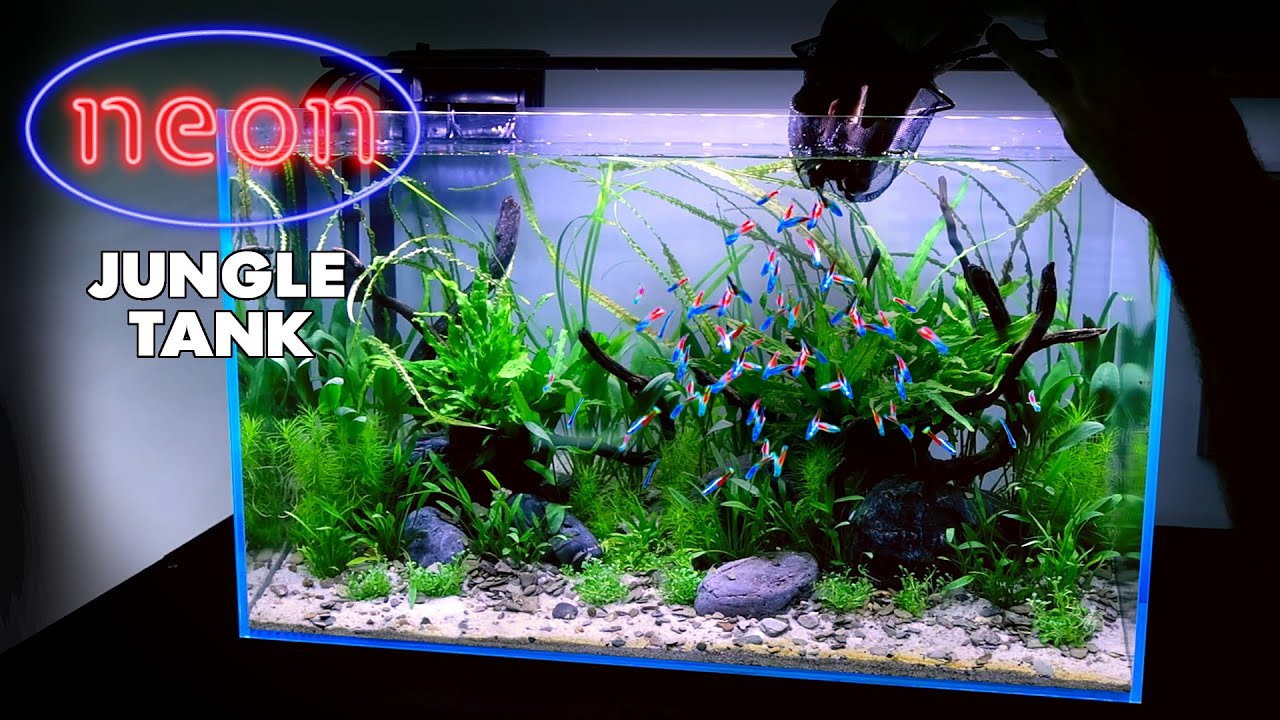This photograph portrays a striking image of a neon jungle-themed tropical fish tank. The tank, which is filled with crystal clear water, is abundantly decorated with artificial plants, decorative gray rocks, and pieces of driftwood that create an enriching jungle-like environment for the fish. The base of the tank is layered with sand and small rocks. Inside, a small school of vividly glowing blue and red neon tetras swim around, their presence further highlighted by the well-lit interior of the tank. The tank's pristine clarity and illumination are set against a darker background, making it the focal point of the image.

A detail that draws immediate attention is the neon sign situated towards the upper part of the image. Encased in a neon blue oval, the word "neon" is displayed in neon red, with "Jungle Tank" written beneath it in large white block letters. There's also a visible hand with a net, interacting with the tank, implying care or maintenance. This vivid and meticulously composed image serves as an advertisement for the strikingly lit and vibrantly decorated Jungle Tank, ensuring the neon tetras and the tank's lush interiors are well-noticed and appealing.